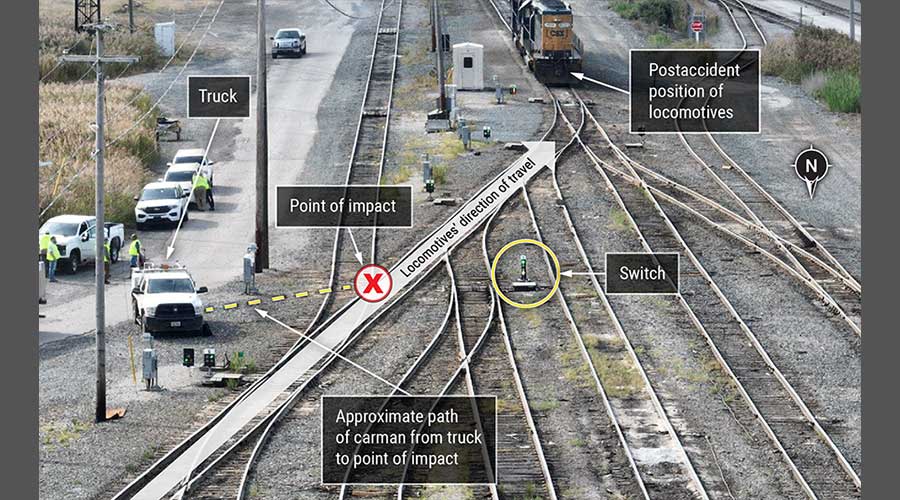This image is a detailed infographic depicting the scene of a railroad accident. Taken during the day, the photograph captures a section of train tracks running mostly north to south, where various elements have been labeled to illustrate the incident. On the left side, there is a paved road with multiple white cars that resemble safety or emergency vehicles. A truck is seen off the road, with an annotation "truck" pointing to it. The truck is connected by a yellow dotted line, labeled as the "approximate path of car man from truck to point of impact," leading to a red X marked "point of impact."

A few individuals in lemon-colored safety vests are standing near the road, presumably inspecting the scene. There is a big white arrow indicating the "locomotive's direction of travel" coming from the bottom left and extending to the top right of the image. The switch on the tracks, circled in yellow, is labeled "switch," and the train is visible at the very top of the image, labeled "post-accident position of locomotives."

Overlaying these annotations are several black boxes with white borders, enhancing key details and directing the viewer's attention to the critical elements of the accident scene. A compass in the right-hand corner indicates the orientation of the image, adding to the clarity and thoroughness of this illustrative graphic.